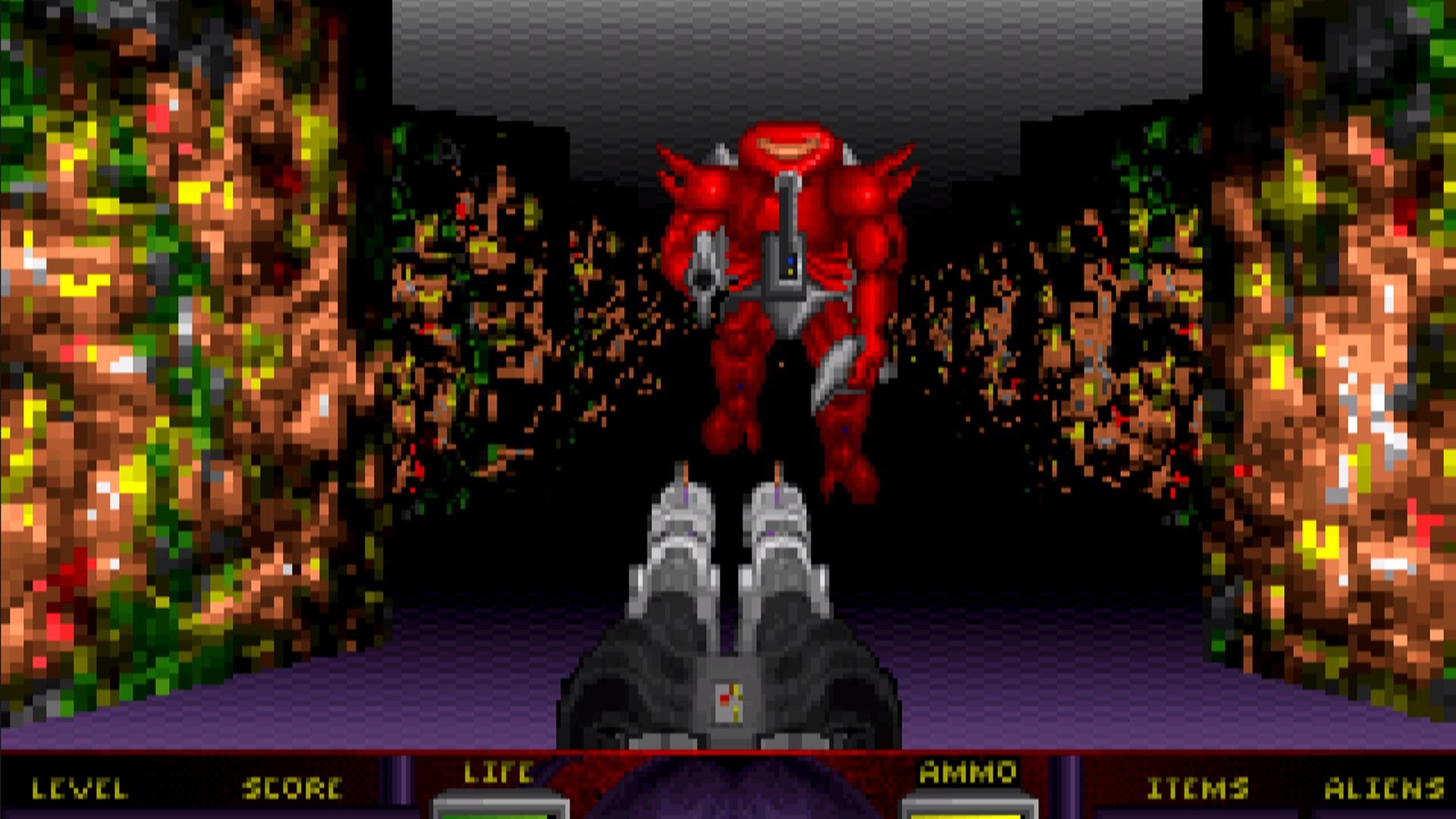The image is a first-person view from a video game, showcasing a highly detailed and intense scene. At the bottom of the screen, game metrics such as level, score, life, ammo, items, and aliens are displayed. Dominating the foreground, a black weapon with twin grayish barrels is aimed directly at an enormous red creature that appears to be a monstrous robot. This creature stands menacingly in the center, adorned with silver armor, including a belt and a leg strap, and holding a large silver gun. The red creature features a solid set of yellow eyes spanning its head, spike-covered shoulders, and muscular arms. The panels flanking the scene are highly pixelated, making any additional details indiscernible, contributing to the overall dystopian and futuristic atmosphere of the game environment.